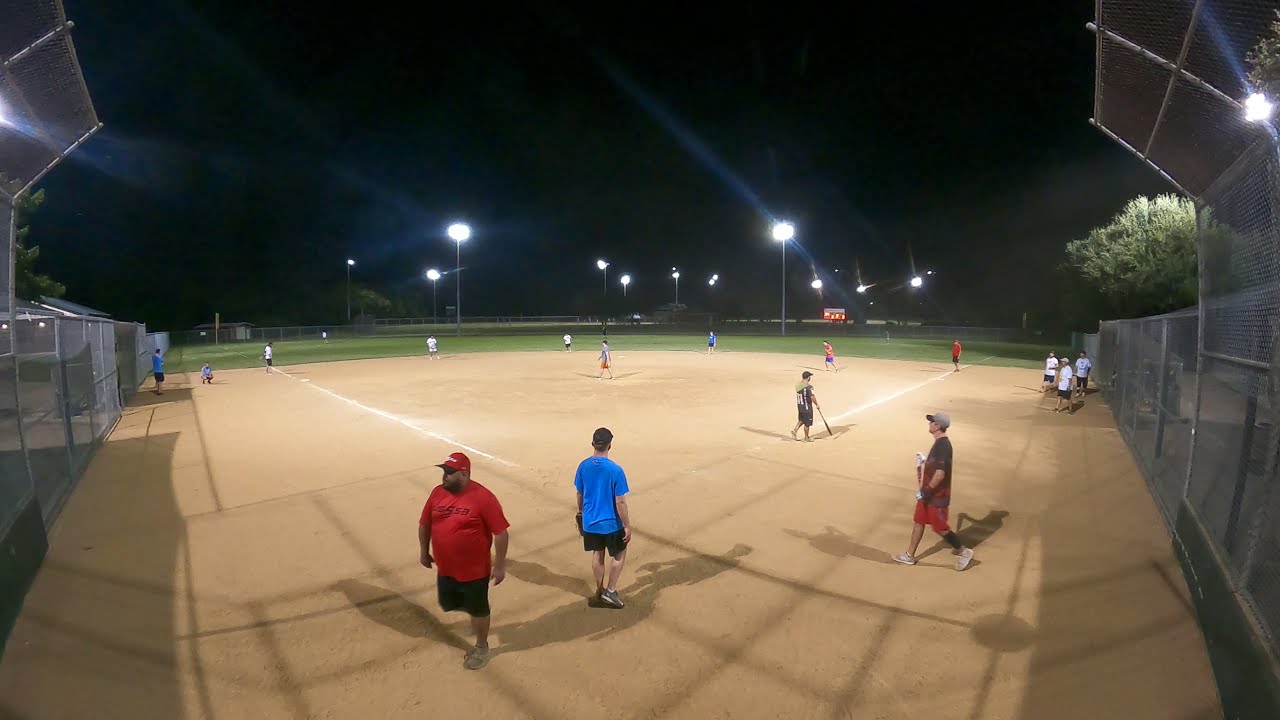This horizontally aligned rectangular image captures a nighttime baseball game. The sky occupies the upper half and is pitch black, sharply contrasting the brilliant illumination cast by numerous light poles scattered around the field. The field itself consists of a brown dirt infield and a distant green outfield with players dispersed throughout. Protective chain-link fencing rises tall on either side, gradually decreasing in height as it extends further into the background.

In the foreground, near the catcher's area, there are two prominent figures. One is a heavier set man in a red t-shirt, red and white baseball cap, black shorts, and sneakers, walking towards the left. The other is a man in a blue t-shirt and black shorts, facing the field. He appears to be the catcher, holding a glove. Off to the right, another man carrying a bat is visible, walking towards the catcher. The entire scene is bathed in the intense glare of the lights, emphasizing the action and ambiance of a nighttime game.